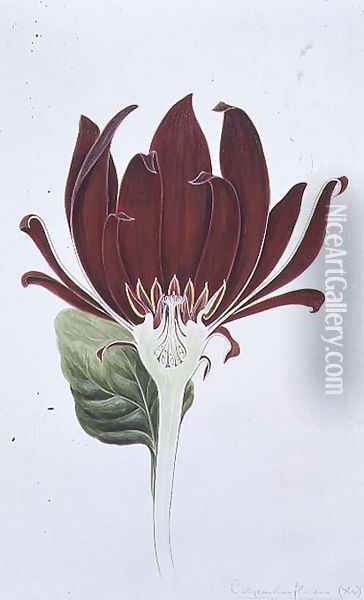The illustration depicts a beautifully detailed flower, resembling a rose petal with a dark burgundy to bright magenta hue. The flower is bisected, revealing its intricate interior structure. It is set against a subtle white to light gray shaded background. The flower's long, white stem supports one prominently detailed green leaf on the left side, enhancing the artwork's realism. Written in vertical white print on the right side of the image is the text "niceartgallery.com," noting the source of the artwork. Additionally, an illegible artist's signature appears in a dark color in the lower bottom corner of the piece.